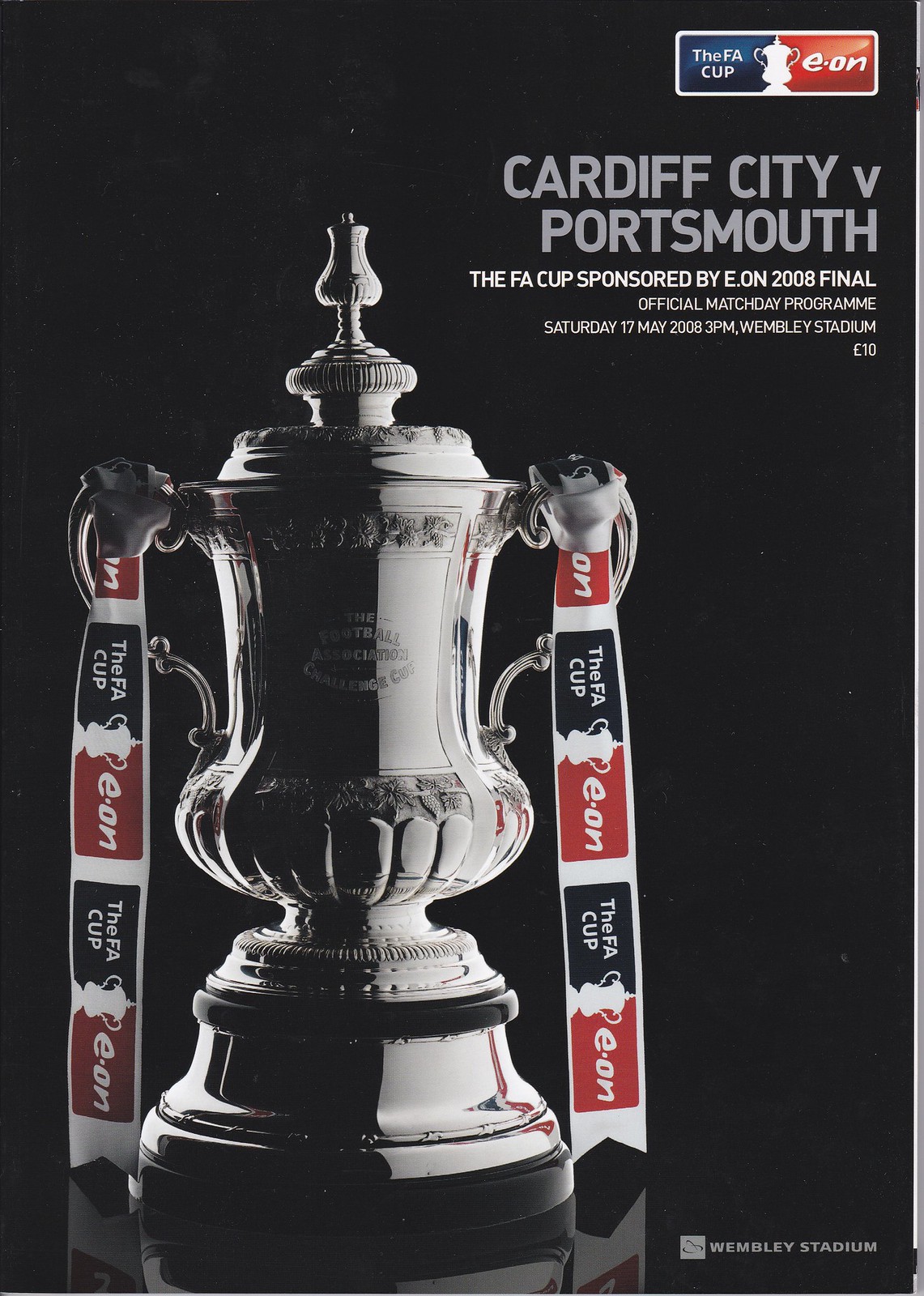This image showcases the official match day program for the 2008 FA Cup Final between Cardiff City and Portsmouth. Dominating the center is a large, gleaming silver trophy adorned with two sashes hanging down from its handles, one on either side. These ribbons are colored red, white, and blue, with inscriptions that read "The FA Cup" and "E.on." The trophy's shiny exterior is dramatically highlighted against a solid black background, with its reflective surface partially illuminated by light, creating an eye-catching visual. 

In the top right corner of the image is the FA Cup logo, featuring a blue, white, and red color scheme with a white trophy outline. Below this, in gray lettering, the match details are clearly inscribed: "Cardiff City v. Portsmouth." Further down, smaller white letters provide more specific information: "The FA Cup sponsored by E.on, 2008 Final, Official Match Day Program, Saturday 17 May 2008, 3 p.m., Wembley Stadium, £10." The bottom right corner also features the Wembley Stadium logo, establishing the venue for this significant sporting event. The overall composition emphasizes the prestigious nature of the FA Cup Final, with every detail meticulously highlighted.